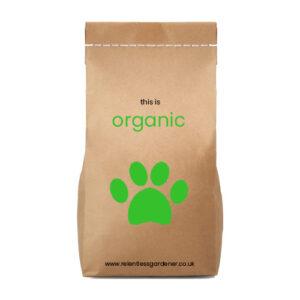The image features a brown paper bag designed for dog food, set against a plain white background. The bag is relatively tall and appears to be of standard grocery store size. Its design includes white stitching approximately an inch from the top, presumably for reinforcement. On the front, the bag prominently displays the word "ORGANIC" in large green letters. Above this, in smaller black letters, the phrase "This is" is printed. Below the word "ORGANIC," there is a large green paw print, emphasizing its suitability for pets. Near the bottom of the bag, a website address is printed, though the exact URL is not specified. The overall presentation suggests a focus on organic and pet-friendly contents, likely making it an appealing choice for conscientious pet owners.